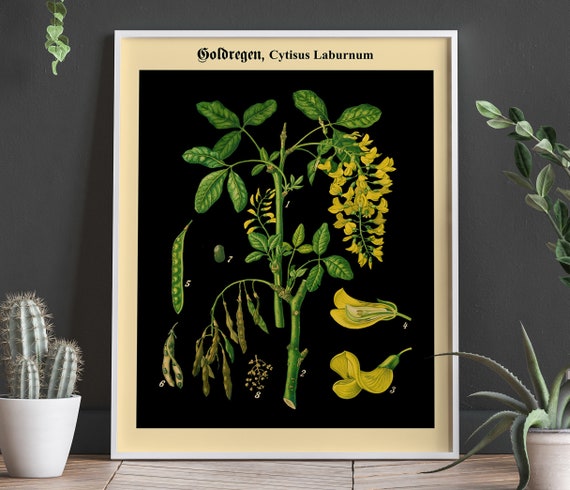The image depicts a detailed painting or illustration of a plant labeled "Goldberg Cytus Laburnum" at the top of the frame. Set against a black background, the plant features numerous green leaves and a green stem but lacks flowers. However, yellow, bell-shaped flowers hang downwards to the right of the plant, with two larger bell-shaped flowers that have fallen to the bottom right. On the left side, dried, green bean-like pods with many smaller pods are visible. Surrounding the framed painting, there is a live potted cactus in a white pot on the bottom left and a long, spiky plant in a beige pot on the bottom right, creating a rich juxtaposition between the painted and real plants. The scene is set against a charcoal gray wall, enhancing the contrast and focus on the central illustrated plant.